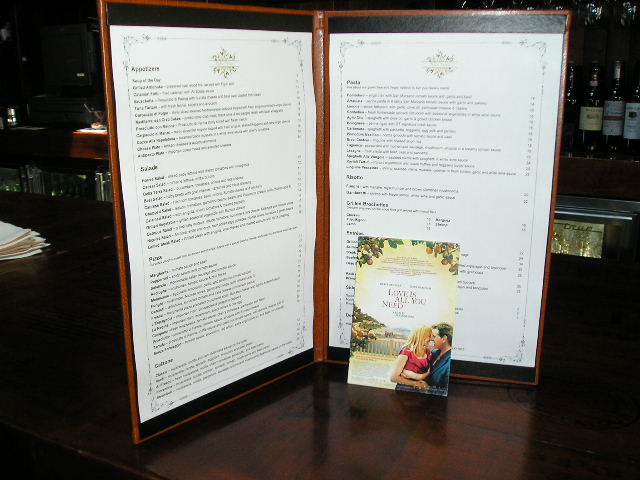This indoor photograph, taken at a cozy bar, captures a detailed view of the bar's wooden interior. The central focus is a brown vinyl menu, elegantly bound with black strips for durability. Resting against the menu is an advertisement, adding a touch of color and information. In the lower middle right section of the image, a refrigerator filled with an assortment of drinks stands behind the bar, complemented by an array of wine bottles displayed on a wooden shelf to the left. On the far left, additional refrigerators are seen, alongside a cash register perched on a wooden cabinet. The bar itself is constructed from rich, polished wood, seamlessly matching the wooden cabinets that store various bar essentials. Adding to the inviting atmosphere, wine glasses hang upside down from the overhead rack in the upper right corner of the photograph, ready for the next pour.